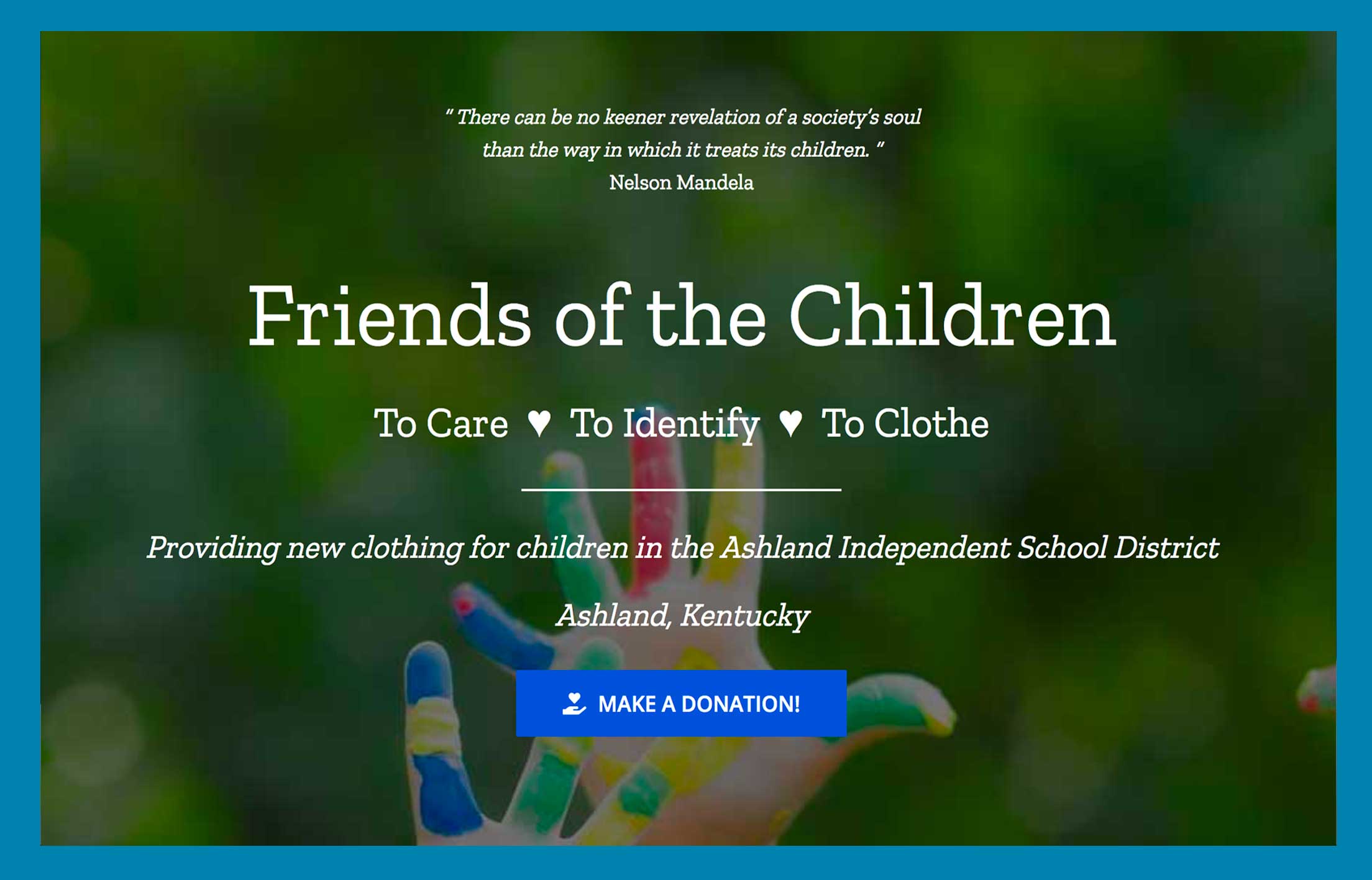The image showcases a screenshot of a website set against a crisp white background. The website is bordered in a medium blue frame, drawing attention to its center where a vibrant, colorful photograph is displayed. The photo captures two children’s hands, palms facing forward. One hand is shown from the wrist up with fingers splayed and painted in various bright colors: the pinky is blue, the ring finger is green, the middle finger is red, and the pointer finger is yellow.

Prominently, atop the image in centered white text, is a profound quote by Nelson Mandela: "There can be no keener revelation of a society's soul than the way in which it treats its children." Below the quote, in bold white text, the website name "Friends of the Children" is displayed, accompanied by the tagline, "To care, to identify, to clothe."

Further down, a descriptive statement reads: "Providing new clothing for children in the Ashland Independent School District." At the very bottom of the central content, a vibrant blue action button is placed, inviting users to "Make a Donation."